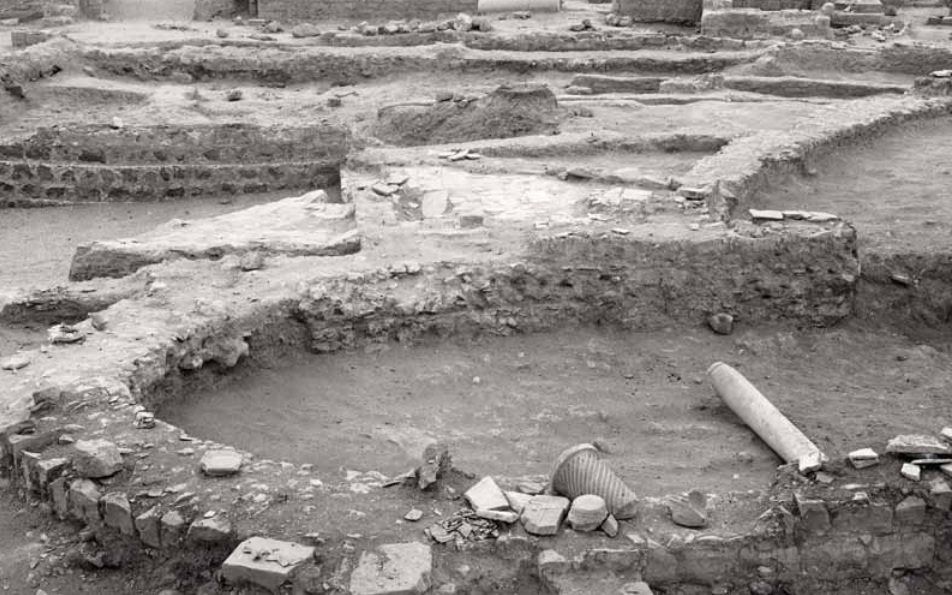This black-and-white photograph, viewed from above at a slight angle, captures an archaeological excavation site. Dominating the foreground is a horseshoe-shaped, shallow indentation encircled by a rough stone wall. Inside this indention, sparse dirt hosts a cylindrical white object, possibly a fallen column segment, extending from the bottom right upward to the left. The area appears largely barren with scattered tools and a basket-like object positioned on the surrounding ledge, which is punctuated with small holes. Around this indention, the terrain is strewn with rocks and debris, creating a textured, muddy appearance. Further in the background, more stone walls rise and curve, delineating another sunken area and suggesting deeper excavation trenches beyond. The distant background reveals additional stone structures, hinting at the remnants of what might have been an old civilization or ruins with parts of buildings still somewhat discernible. The image's monochromatic palette accentuates the uniform grayness and texture of dirt and stone, imbuing the scene with a stark, timeless quality.